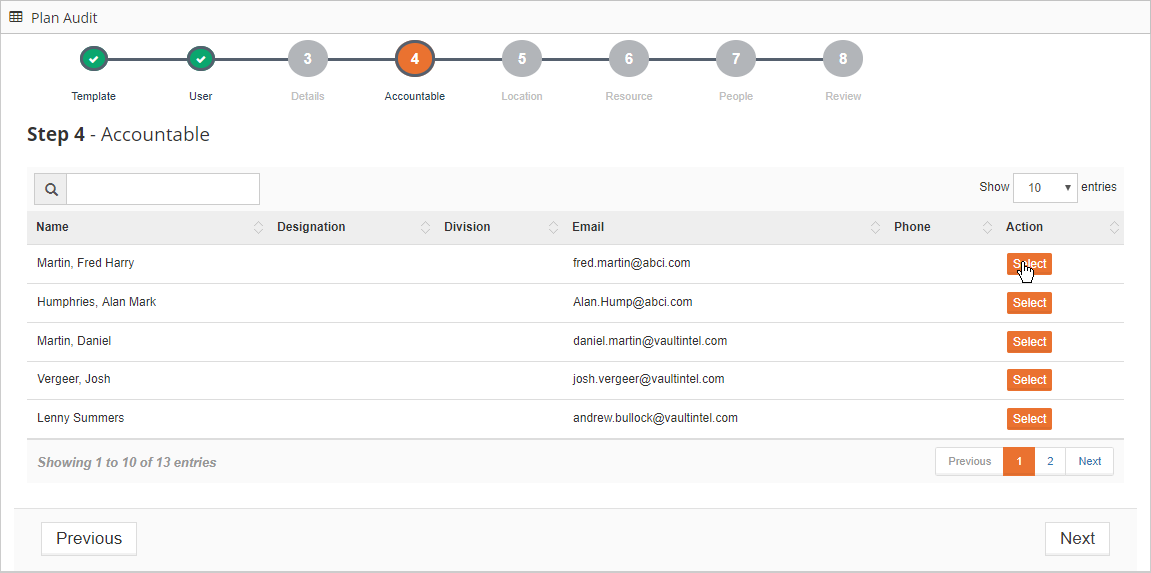The image displays a detailed audit plan workflow on a computer screen. The top section of the screen features a progress tracker depicted through a series of connected gray steps numbered from 1 to 8. Within this tracker, steps are represented by circles, with the first two steps highlighted in green circles containing white checkmarks, indicating completion. These initial steps are labeled "Template" and "User."

As the steps progress, step 3 appears as an incomplete task, shown as a gray circle marked with a white number "3" and labeled "Details." Moving to step 4, the circle transitions to orange with a number "4," indicating the current active step labeled "Accountable." Below "Accountable," the subsequent steps include step 5, "Location," step 6, "Resource," step 7, "People," and step 8, "Review," all of which remain in gray, signifying pending completion.

Beneath the progress tracker, the page lists a series of names: Martin, Fred, Harry, Humphreys, Alan, Mark, Martin, Daniel, Vern, Josh, and Lenny Summers, presumably team members involved in the audit process.